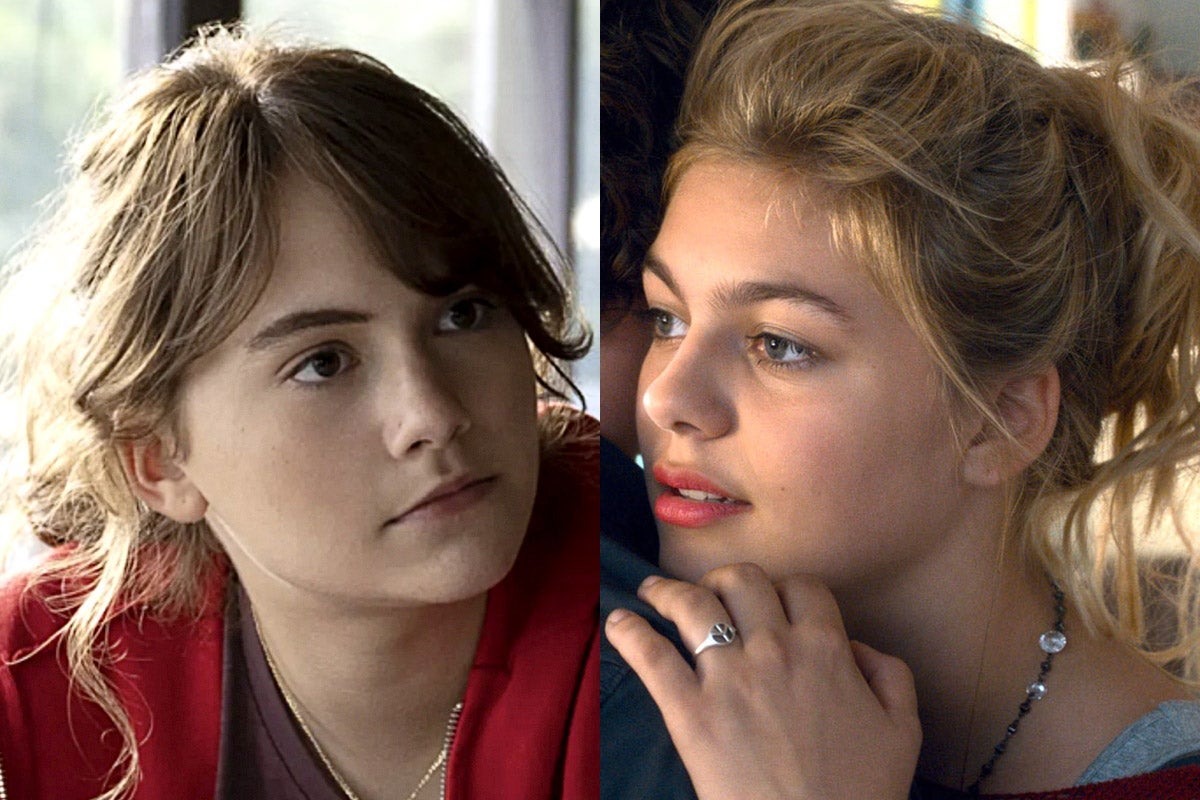The image comprises two side-by-side photographs of two women around their early to mid-twenties, each occupying half the frame. The photograph on the left showcases a woman with dark brown hair and eyes, wearing a red jacket over a brown shirt. She appears plain and makeup-free, with a concerned or focused expression as if listening intently. Her surroundings and general aesthetic seem more subdued and serious.

In contrast, the photograph on the right features a woman who might represent the same individual at a different time or a different woman altogether. Her lighter blonde hair is styled in a ponytail, and she has noticeable makeup, including salmon-pink lipstick. She accessorizes with a peace sign ring and a necklace with clear crystal beads. Her expression is dreamy and content, suggesting she might be embracing someone, with a general air of happiness and daydreaming. The colors in this photograph appear more vibrant and lively, highlighting her happier demeanor. The stark difference in emotions and presentation between the two images suggests a possible narrative of change or contrast, perhaps indicative of a TV show or movie.